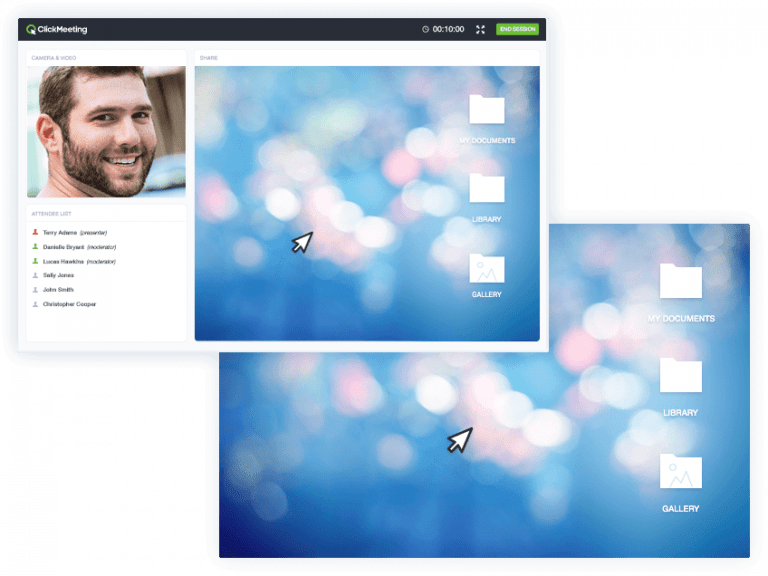This image, sourced from the website ClickMeeting, showcases two overlapping interface screens. The top screen is positioned on the upper left-hand side, while the larger, slightly obscured screen is at the bottom right. On the top screen, the ClickMeeting logo, a green circle, is distinctly visible on the upper left. On the upper right-hand corner, there is a noticeable green button and a timer displaying "10 minutes." Dominating the left-hand side of this screen is a close-up photograph of a smiling man with a beard and brown hair. His body is oriented toward the right, but his face is turned towards the camera. Below the man's image, a vertical menu bar is seen. The second, larger screen located at the bottom right serves as a subtle backdrop to the first, providing additional context to the visual representation of the ClickMeeting interface.